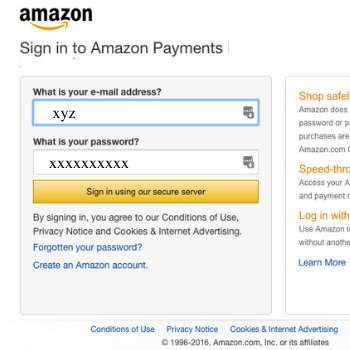This cropped screenshot captures the sign-in interface for Amazon Payments, presented on a clean, white background. Prominently positioned at the top left is the familiar Amazon logo. Below the logo, large black letters command the user to "Sign in to Amazon Payments."

Dominating the center of the interface is a sizable grey box. The first section of this box poses the question "What is your email address?" in small black text, accompanied by a large input field below, which contains the placeholder text "XYZ." Further down, another query, "What is your password?" is shown in the same small black font. Beneath this, the password field displays a series of X's indicating hidden characters.

At the bottom of the grey box, a substantial yellow button invites users to "Sign in using our secure server," the text centered in small black letters. Directly underneath this button, a disclaimer informs users that by signing in, they agree to Amazon’s Conditions of Use, Privacy Notice, and policies on Cookies and Internet Advertising.

Toward the bottom left of the grey box, two blue hyperlink options are offered: "Forgotten your password?" and "Create an Amazon account." On the right edge of this section, a partial white box is visible, revealing only its far left side due to the cropping. Inside this cropped white box, category headings are highlighted in orange with accompanying descriptions in small black print, concluding with a "Learn more" link at the bottom in blue hyperlink font.